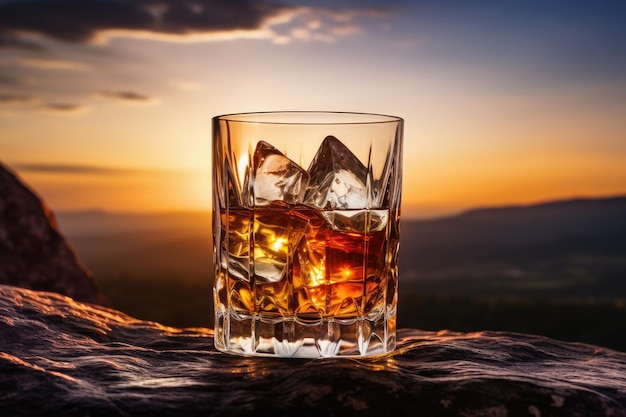A glass with a thick base, typically used for alcoholic drinks, sits on a rocky, uneven surface in front of a picturesque landscape. Filled with ice cubes almost to the top and containing an amber liquid assumed to be alcohol, the glass is placed prominently against a backdrop of a sunset or sunrise. The sun is partially visible on the horizon, casting warm orange, brown, and yellow hues through the liquid and ice. The sky, tinged with the colors of dusk or dawn, features scattered clouds primarily on the left side, while the ground below appears to be a mix of blurred mountains, valleys, and possibly a city area. The overall scene offers a serene yet dynamic composition, with the wavy, natural landscape supporting the stability of the glass.